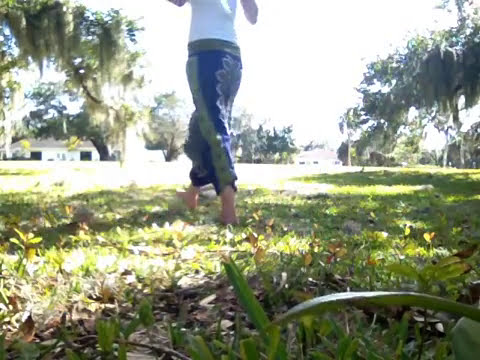The photo captures an outdoor scene from ground level, focusing on a person walking away from the camera. The image's foreground prominently features green and brown grass, detailing the texture close to the camera. The barefoot individual, appearing slim, is wearing decorated capri-length blue and green pants and a white shirt. The camera angle cuts off the top part of the person, directing attention to their lower half as they move towards a distant, sunlit building. Tropical trees frame both sides of the scene with their branches arching into the frame, casting shadows on the grassy lawn. The sky in the background is overwhelmingly bright, displaying as a solid expanse of white light, enhancing the overall glare and making the atmosphere appear sun-drenched and vividly illuminated. In the distant background, a white house on the left and another on the right are faintly visible through the glare, anchoring the bright horizon behind the trees.